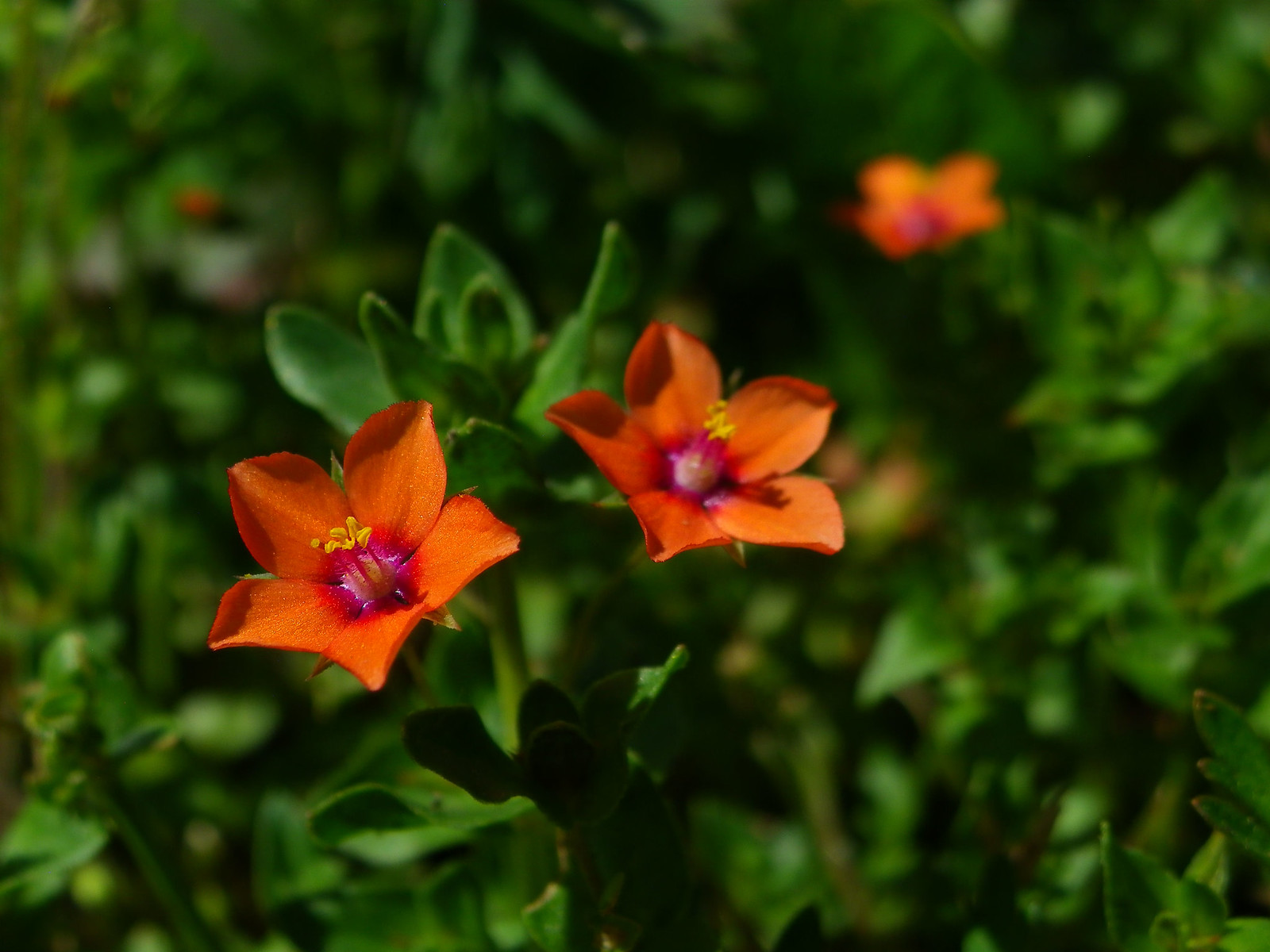This is a detailed photograph capturing the striking beauty of two prominent orange flowers with radiant green foliage in the background. The flowers, which are likely daffodils, each display five slightly triangular petals that transition from a vivid orange on the edges to a rich purple towards the center. Each center also features yellow-tipped stems protruding and small dashes of white, adding intricate detail. A third orange flower can be seen blurred in the background, enhancing the depth and overall composition of the image. The lush green leaves surrounding the flowers are round and robust, with a couple positioned below and behind the blossoms. Set in a bright daytime outdoor environment, possibly a garden or forest, the backdrop is a tapestry of vibrant green shrubbery. The photograph's focus on the flowers against a blurred, verdant background creates a harmonious and picturesque scene.